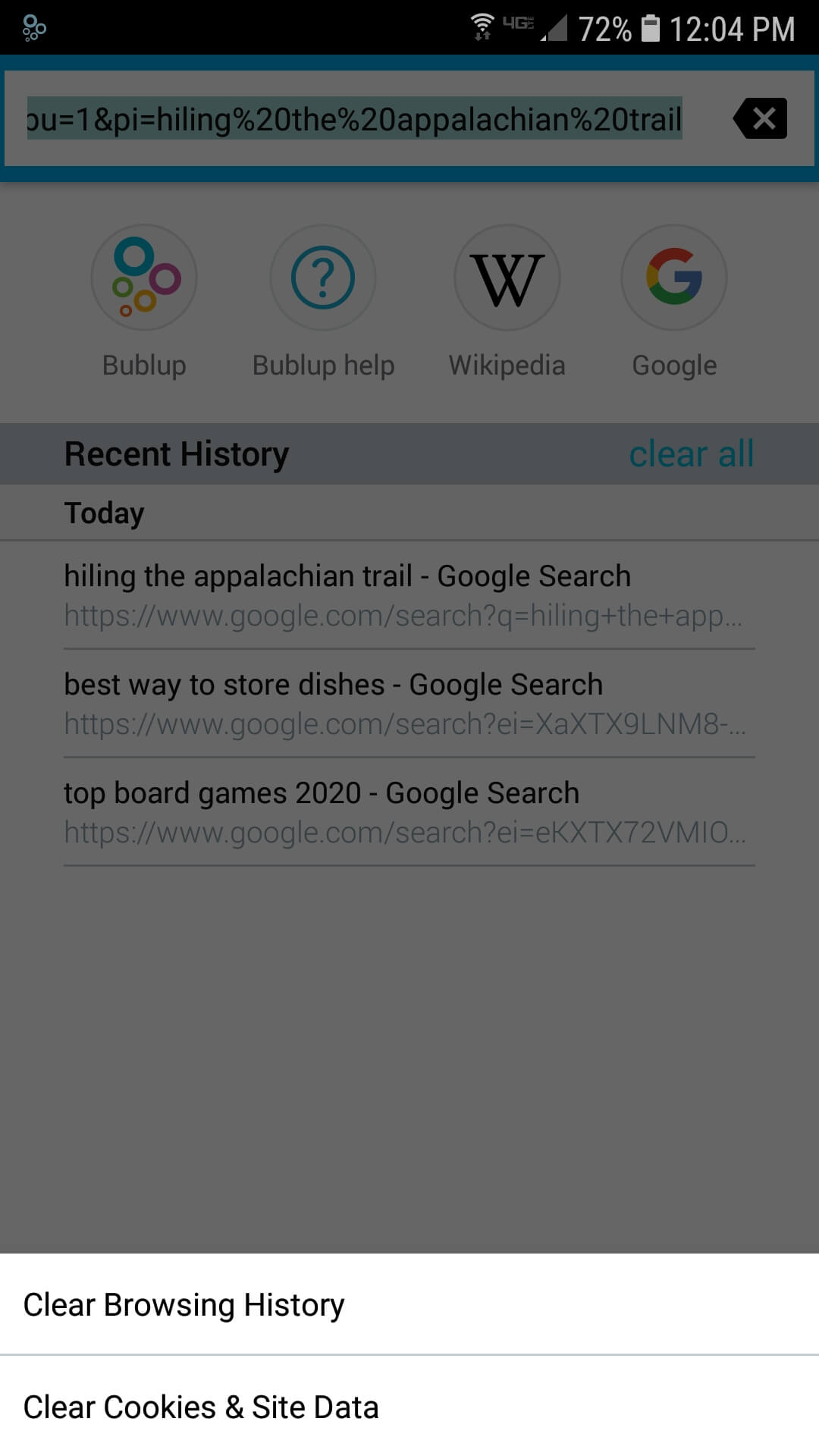The image displays a smartphone screen open to an unfamiliar web browser interface. The browser's address bar is active, with the previous URL highlighted, indicating readiness for a new web address to be entered. No new URL has been typed yet. Beneath the address bar, there are several favorite sites and apps displayed with their respective icons: Bubble Up (stylized as "Bublup"), Wikipedia, and Google. The Bubble Up icon depicts various-sized, colorful bubbles. Below this section, the screen shows a list of recently visited sites labeled "Recent History." The entries include "Hiking the Appalachian Trail," "Best Way to Store Dishes," "Top Board Games 2020," each accompanied by their respective URLs. Additional browser options at the bottom include a "Clear All" button beside the favorites and a "Clear Browsing History" button alongside a "Clear Cookies" option, suggesting privacy management features. The overall design features a clean, white background with predominantly black text for legibility.